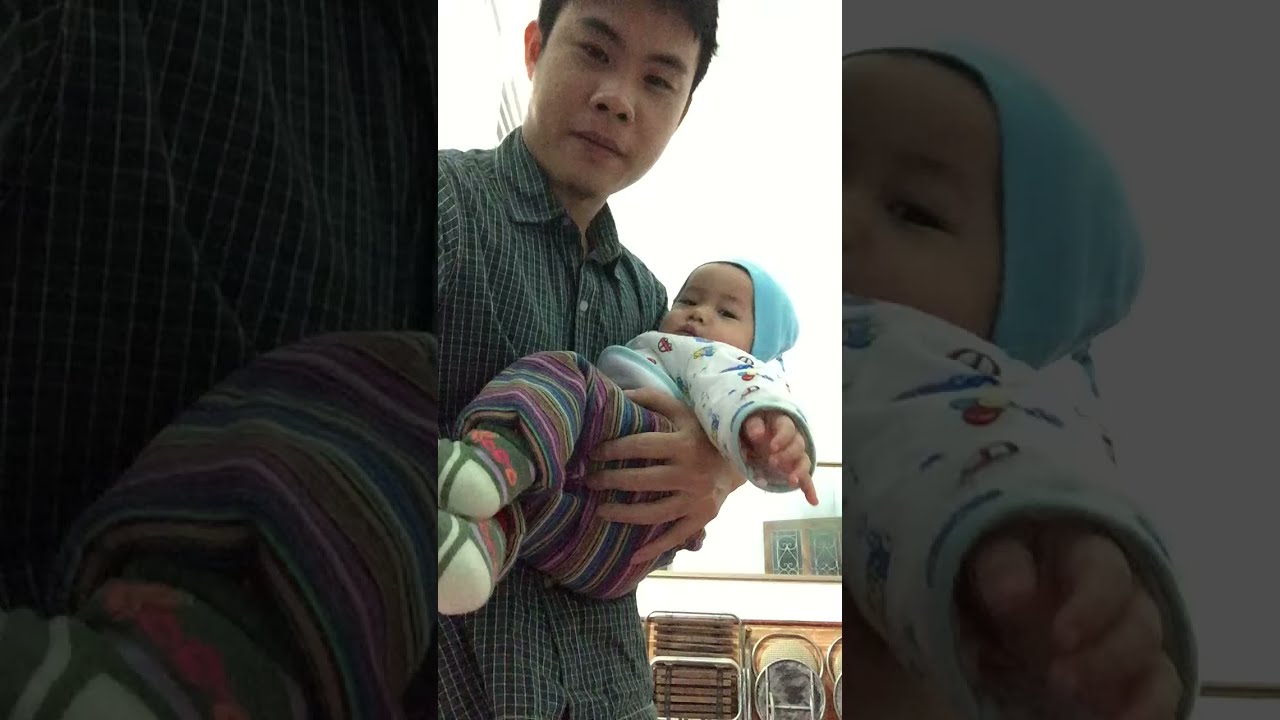In this detailed photograph, we see an Asian man standing in the center of a room with tall white walls and a high ceiling adorned with green designs. He is dressed casually in a black-and-white striped collared short-sleeve shirt and black pants. The man is holding a baby, who is bundled comfortably in his arms. The baby, who appears quite large, is wearing a blue beanie, a white jacket, colorful pants, and is wrapped in a red towel. Both the man and the baby are smiling and looking content.

Surrounding them, the room is sparsely decorated but contains several notable features. To the left, near the ceiling, there is a vent, and further down is a window. Dominating the ceiling is a fan. Behind the man, there's a baby trailer and possibly a mirror reflecting some part of the room. On the right side of the photograph, there are some chairs against the wall. The bottom of the photo shows some shelving and a stroller in the bottom left corner. The colors in the room include shades of green, blue, brown, gray, tan, white, light blue, and light green, adding a subtle variety to the otherwise simple setting. The overall ambiance suggests it's daytime and could very well be inside someone's living room or the baby's nursery.